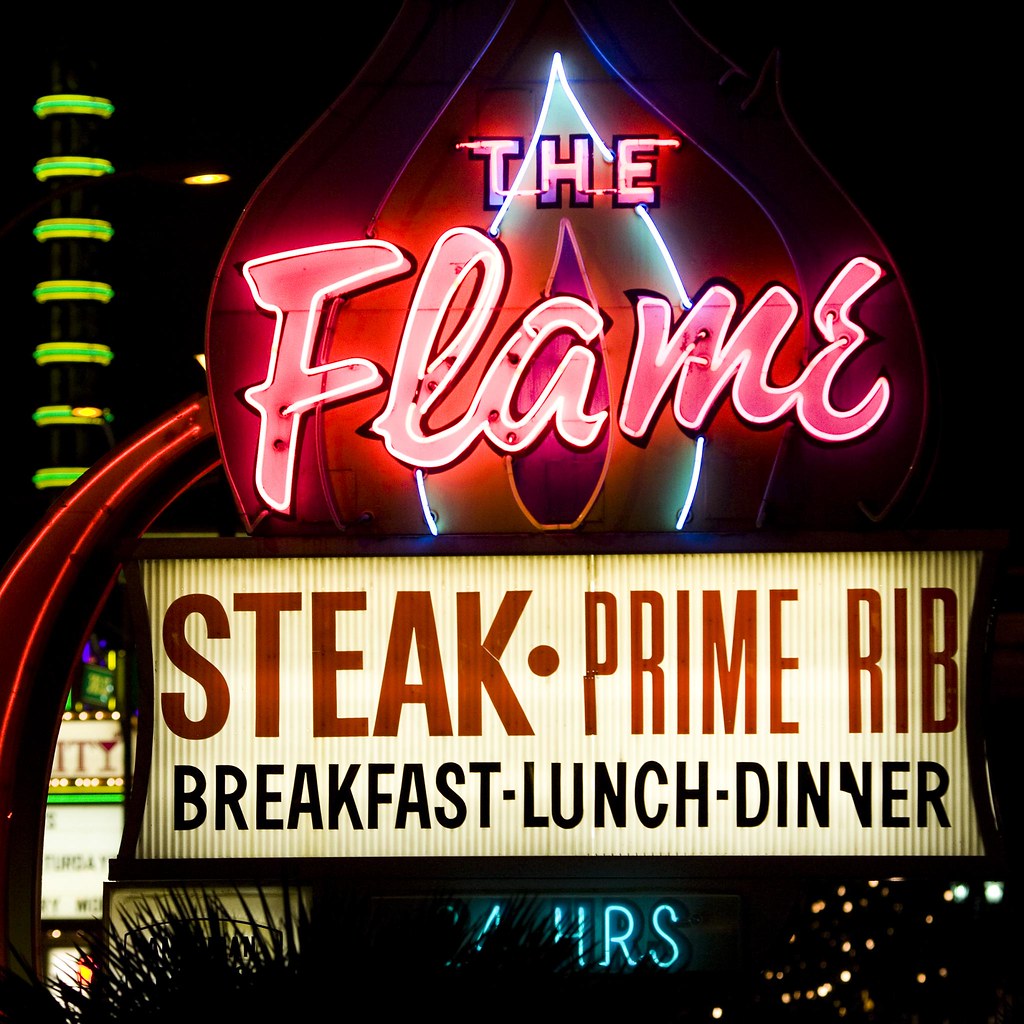This photograph captures a neon sign for a restaurant taken at night, set against a dark backdrop. The top portion of the sign reads "The Flame" in vivid pink neon, with a stylized candle flame depicted behind it in pink and red hues. Below this, a rectangular white board features "Steak, Prime Rib" in bold red letters, while underneath that are the words "Breakfast, Lunch, Dinner" in black. At the bottom, partially obscured by foliage, a blue neon sign displays "24 Hours," though only "HRS" and part of a "4" are visible. In the upper left-hand corner, a nearby structure showcases neon yellow and green rings, possibly part of a hotel or similar building, indicative of a bustling downtown area. The overall scene, with hints of other neon signs in the background, suggests a lively nightlife environment, possibly in a place like Las Vegas.